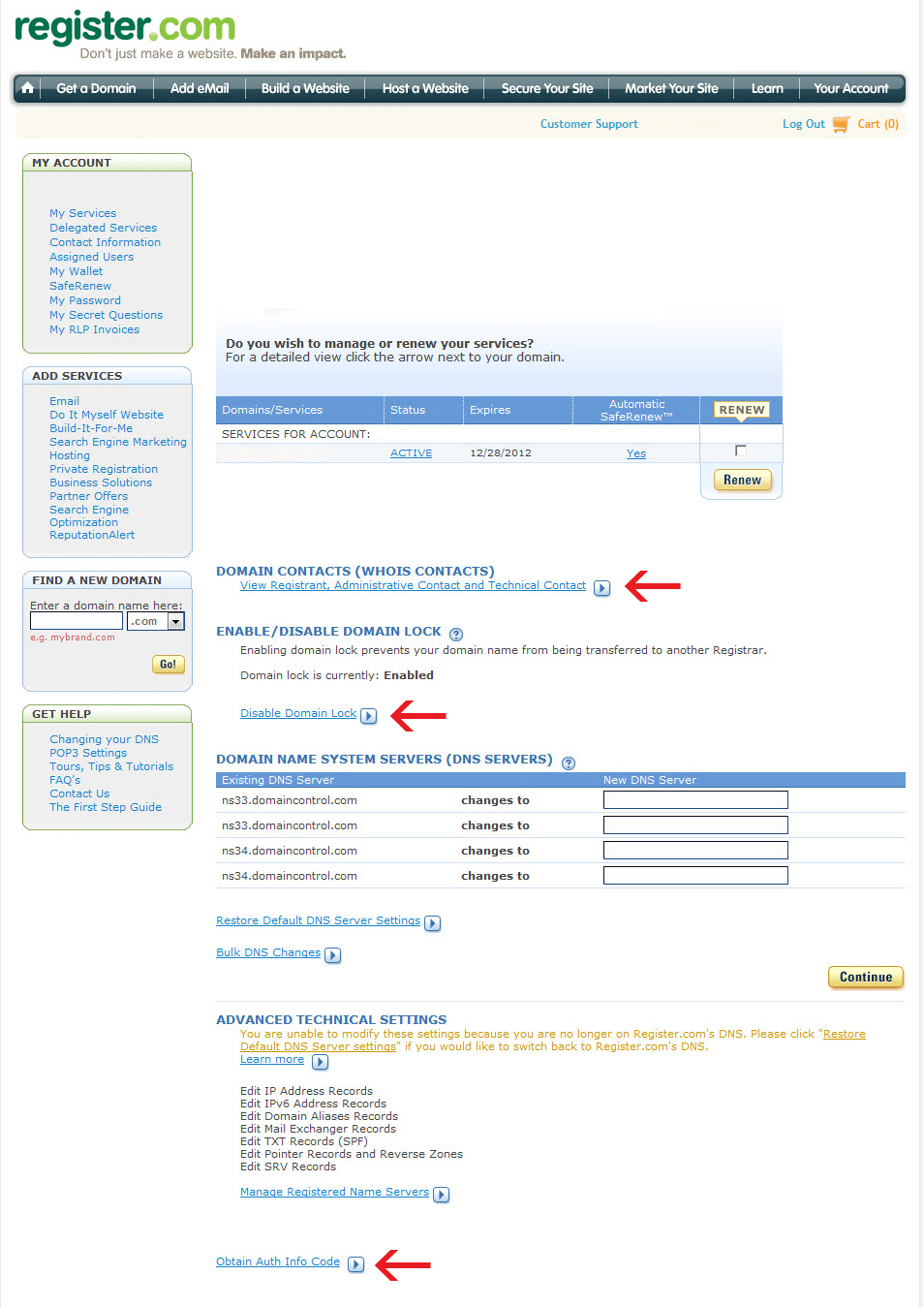**Caption:**

On the top left of the image, there is a green text that reads, "register.com. Don't just make your website, make an impact." Below this, a series of tabs are displayed against a black background with white text. The tabs, from left to right, include: Home, Create a Domain, Add Email, Build a Website, Host the Website, Secure Your Site, Market Your Site, Land Your Account. 

At the top right, there are options for "Your Account," "Logout" in blue, and "Cart" in orange. To the left of "Logout" is "Customer Support" also written in blue.

On the left side of the image, there are four sections:
1. **My Account** (text in blue): Includes sub-options like My Services, Delegated Services, Contact Information, Assigned Users, My Wallet, Safe Renew, My Password, My Secret Questions, and My RLP Invoices.
2. **Add Services**: Includes Email, Do It Myself Website, Build It For Me, Search Engine Marketing, Hosting, Private Registration, Business Solutions, Partner Offers, Search Engine Optimization, and Reputation Alert.
3. **Find a New Domain**: A text box to type the domain name (example: express4debt.com) followed by a yellow "Go" button.
4. **Get Help**: Includes options like Change Your DNS, POP3 Settings, Tool Tips and Tutorial, FAQs, Contact Us, and The First Step Guide.

On the right side, the text asks, "Do you wish to manage or renew your services?" and prompts for a detailed view by clicking the arrow next to your domain. Below this, it shows the domain or services status - the domain is active, Safe Renew is enabled, and there is a yellow "New" button.

Further down, labeled sections include Domain Contact, WHOIS Contact, Services Administration, Administrative Contacts, and Technical Contacts, with a red arrow pointing to the text. Below, it mentions the option to "Enable or Disable Domain Lock," explaining that enabling it prevents the domain name from being transferred to another registrar. The domain lock is currently enabled, with another red arrow pointing to this part.

At the bottom, DNS-related settings are detailed, including a table for DNS servers, the option to Restore Default DNS Server Settings, and advanced technical settings. It notes that modifications are restricted if you are no longer on register.com DNS, advising to revert to default settings if desired. Additionally, there is an option to "Edit IP Address Record."

Finally, the manage settings section features options like Manage Registrars, Name Servers, and Obtain Authorization Code, with yet another red arrow pointing to these options.